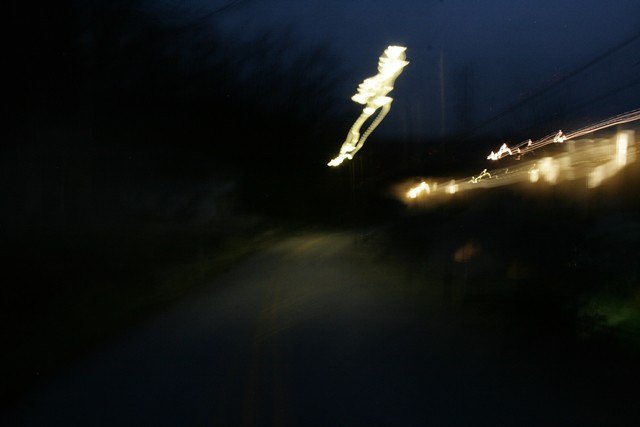The image depicts a blurry, nighttime scene along a dimly lit rural road. The image is characterized by motion blur, suggesting it was taken with a long exposure. A faint, streaky light, possibly from a lamppost, extends across the top middle portion of the image, appearing almost skeletal in shape. This light creates an abstract, bright white burst. To the right, multiple white squiggles of light streak across the image, adding to the sense of movement.

Below, the road, marked by solid yellow lines, is partially visible amidst the darkness. The road is flanked by green shrubbery and grass, with more trees discernible on the left side. Black connecting cables stretch across the scene, adding to the rural ambiance. The background shows hints of a blue night sky interwoven with patches of black, emphasizing the dark, nighttime setting. The overall image gives an impression of a blurry, dynamic, and somewhat eerie roadside nightscape.